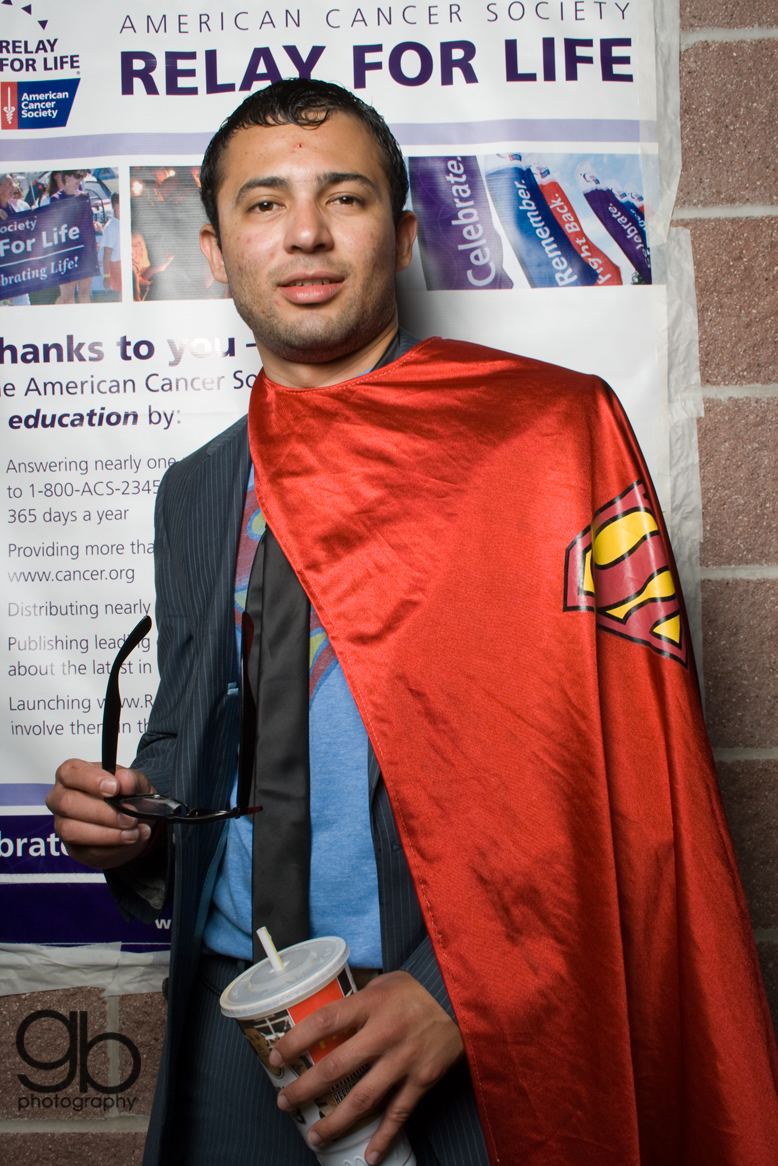In this photograph, a tan man with short, slightly curly dark hair stands facing the camera. He has a slight smile on his face and appears to be South American in descent. He's dressed in a blue-gray suit with a black tie and a blue shirt underneath the jacket. Draped over his left shoulder is a distinctive Superman cape, featuring the iconic red 'S' against a yellow background. The man's right hand holds a pair of sunglasses while his left hand clutches a disposable fast food drink cup with a plastic lid and a straw. He stands in front of a stone or brick wall, with gray grout contrasting against the reddish light brown bricks. Behind him, a poster announces a Relay for Life event, associated with the American Cancer Society. At the bottom left of the image, there's a watermark that reads "GB Photography" in black letters.